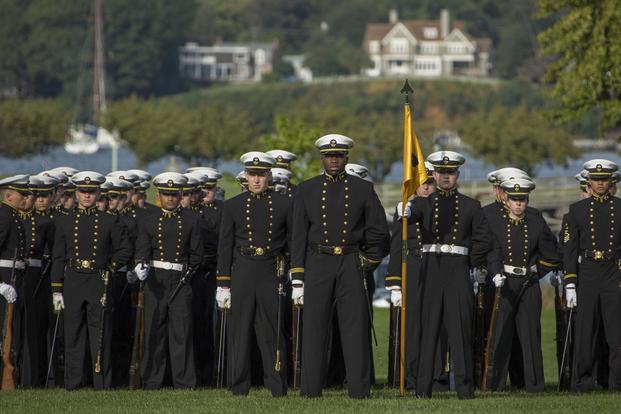The image depicts a military parade or formation practice, seemingly a naval event. At the forefront, numerous young men dressed in striking uniforms stand shoulder to shoulder in neat rows. Each uniform consists of a black long-sleeved coat adorned with two rows of gold buttons, black pants, white gloves, and white, brimmed military hats featuring a black bill and a golden rope encircling the hats with a central gold emblem. A commanding figure, potentially the troop leader, stands prominently in the middle, accompanied by another individual holding a yellow flag. The scene unfolds on a lush, green field bordered by several bushes. In the middle ground, a calm body of water, possibly a river or bay, lies adjacent to the field, supporting a tall sailing ship. This vessel is slightly blurred but adds a nautical charm to the scene. Further back, on a slight hill, stand two large, opulent houses painted in white, gray, and brown, completing the picturesque background. The image resonates with the solemnity and precision of a military event, accentuated by the vivid colors of the uniforms, the yellow flag, the greenery, and the serene blue waters.